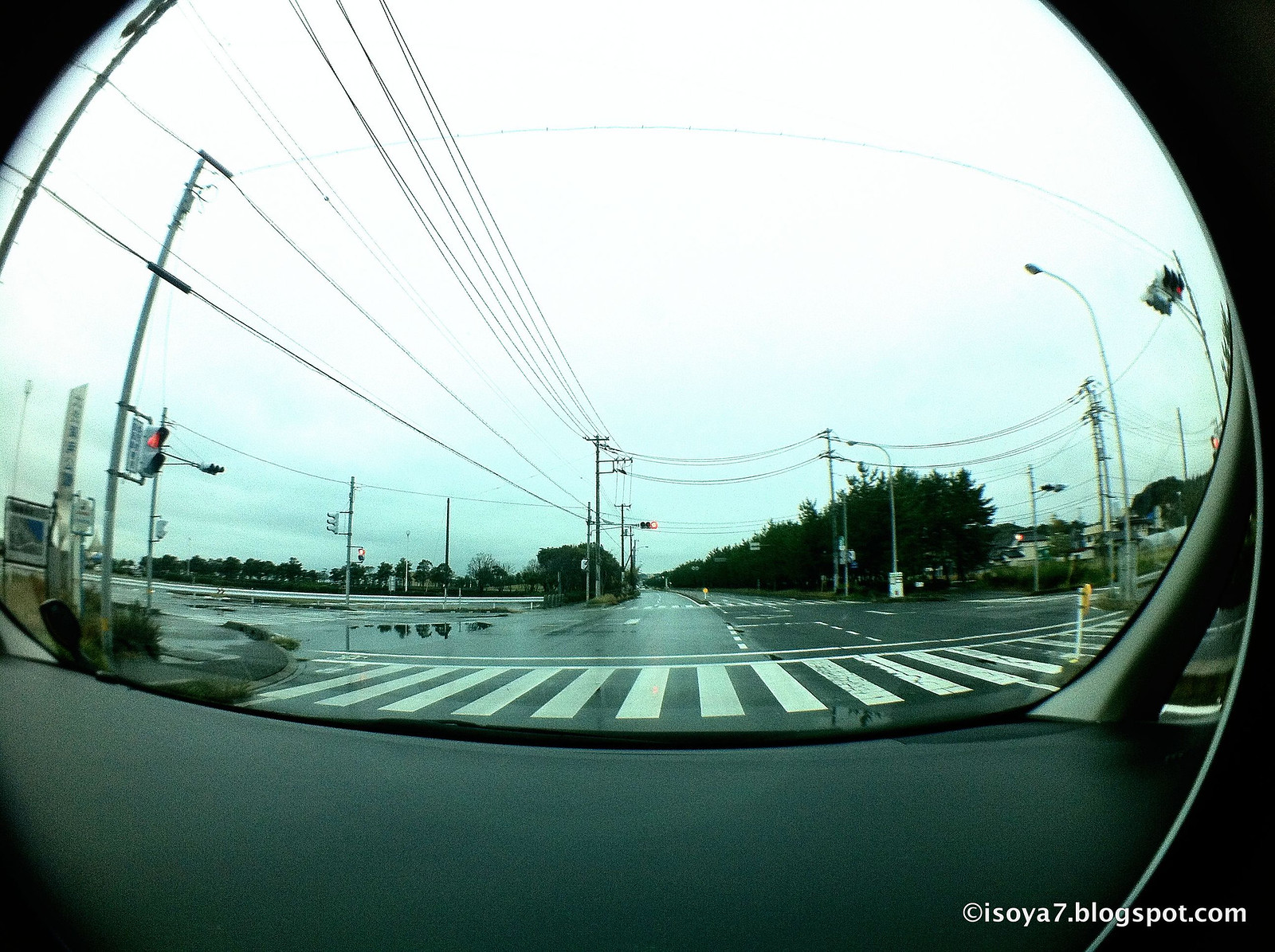The image, captured with a fisheye lens, showcases a street scene with a distinctive fishbowl effect, giving it a wide-angle perspective. The foreground prominently features a crosswalk spanning the width of the street, set against a backdrop of black asphalt. Flanking the crosswalk on either side are poles and traffic lights. To the left, a traffic light with two lights and visors displays a red signal at the top. Behind this light, a small billboard and a rectangular sign are visible, adding layers of depth. The scene is interspersed with several telephone poles and wires crisscrossing above. In the background, another traffic light also shows red, contributing to the urban tapestry.